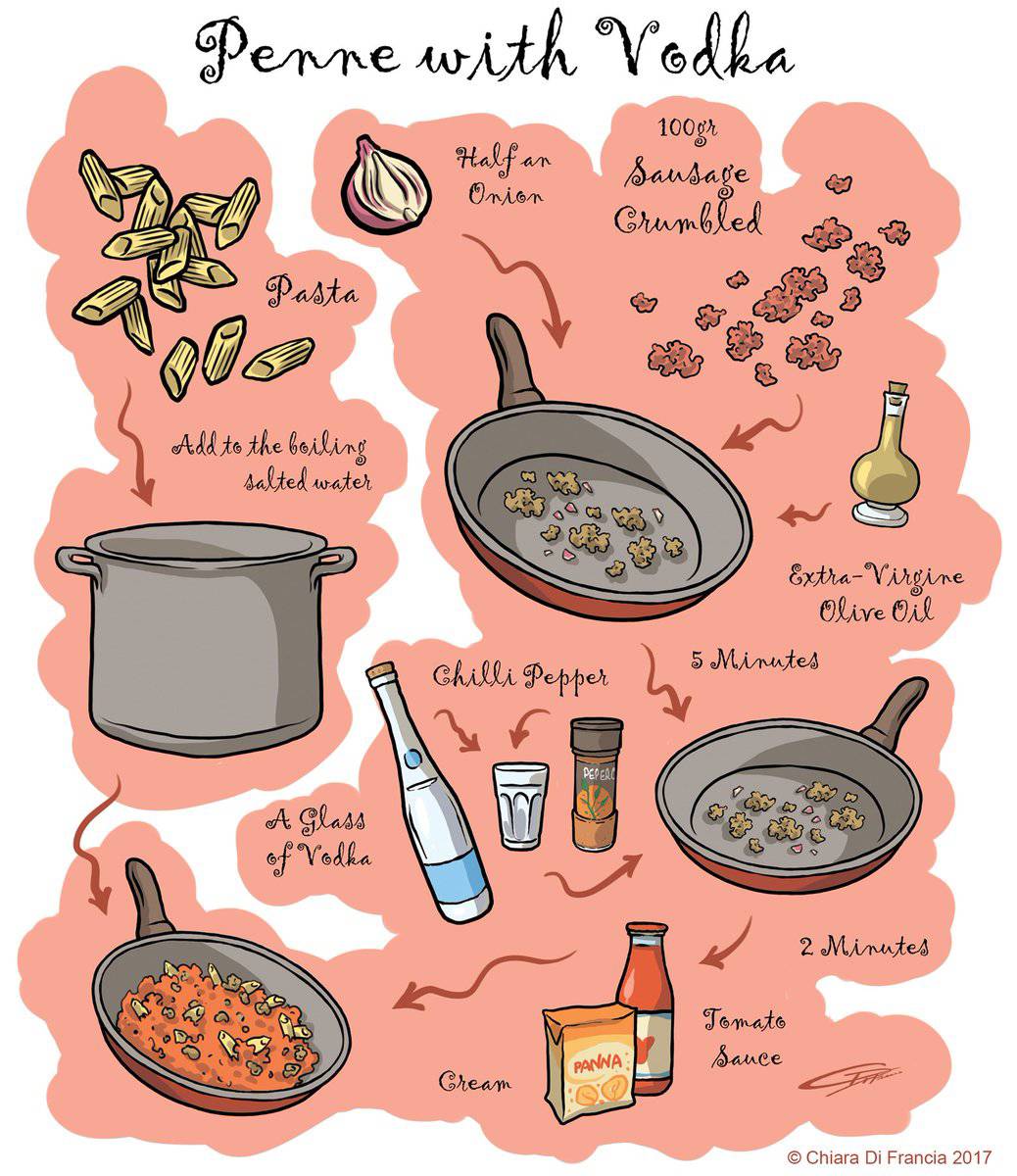This is a comic book-style illustrated recipe for "Penne with Vodka," set against a white background with cartoon graphics and black cursive text. The image is divided into sections with pink cloud-like shapes containing the step-by-step instructions. At the top, the title "Penne with Vodka" is prominently written in loose script. The upper left features a large gray cooking pot with yellow penne pasta dramatically falling into it. To the right, cartoon depictions of ingredients include a yellow onion, red sausage crumbles, and a bottle of yellow liquid, likely olive oil. Arrows connect these ingredients to a frying pan with a gray center and red rim. Below these, additional arrows point to a white salt shaker and a tall red bottle of tomato sauce. Detailed text, although small, describes the process: starting by adding penne pasta to boiling salted water, cooking half an onion and 100 grams of sausage crumbles in olive oil for five minutes, then adding chili pepper and a glass of vodka to cook for another two minutes before finishing with tomato sauce. The finished dish is illustrated in the lower left, showing the combined ingredients in the frying pan. Finally, a copyright note in the bottom right reads "© Chiara Di Francis, 2017."